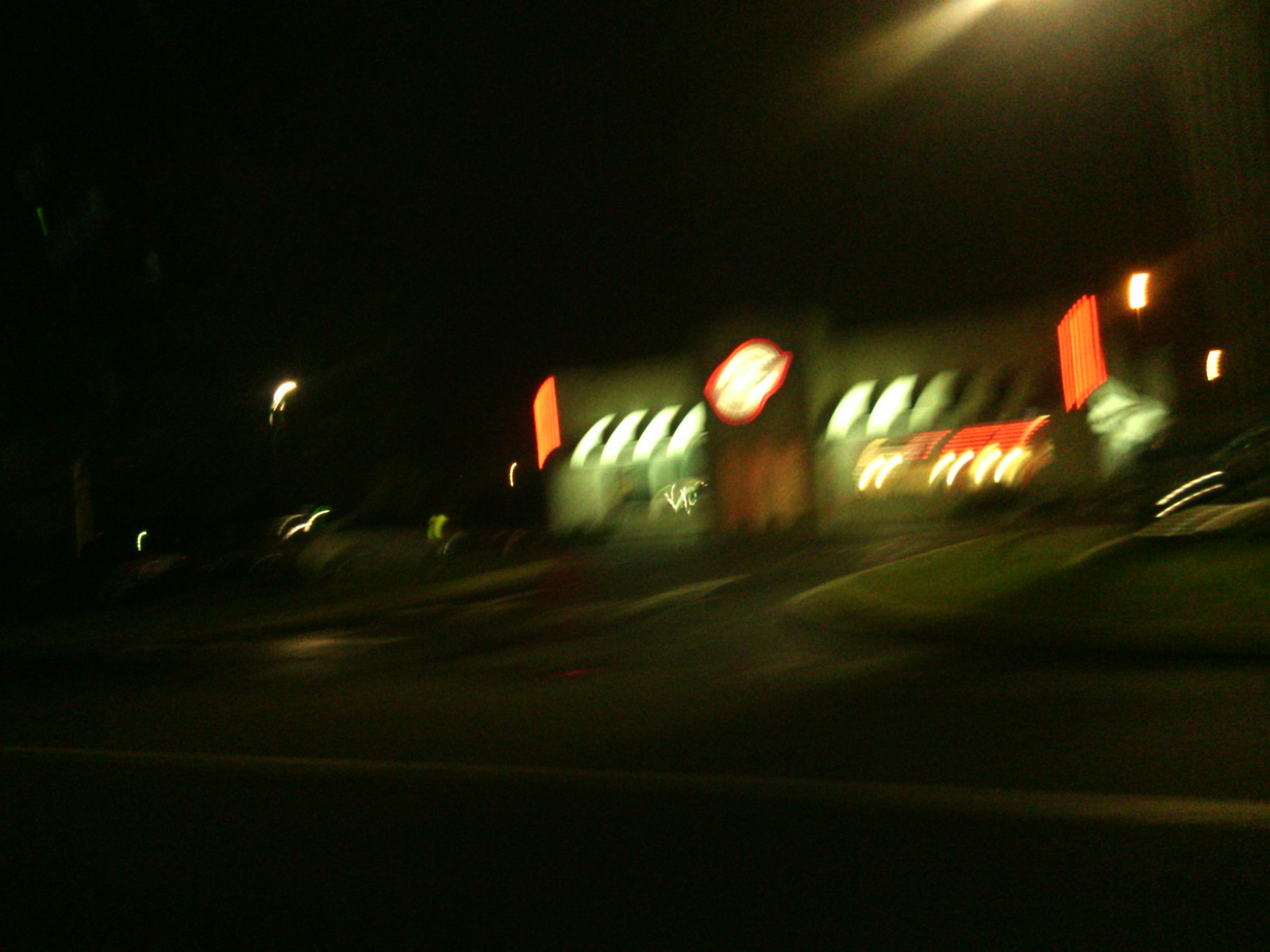This is a color photograph taken at nighttime, characterized by dim and moody lighting. Instead of the usual pitch-black sky typical of night scenes, both the sky and the road are rendered in a dark, greenish-gray hue, contributing to an almost surreal atmosphere. The lower portion of the image clearly depicts a road, identifiable by a central dividing line, which under the low-light conditions appears as a dull greenish color.

Dominating the right-hand side of the frame, a fast-food restaurant is discernible despite the blurriness of the image. The establishment is well-illuminated, contrasting sharply with the surrounding darkness. Two vivid orange signs flank either side of what seems to be the main entrance, casting a welcoming glow. Above the entrance, there's a noticeably blurry sign that likely displays the restaurant's logo, which is an indistinct yellow and orange oval. Despite the lack of sharpness in the image, the light from the restaurant provides a focal point, drawing the viewer's attention amidst the dim surroundings.